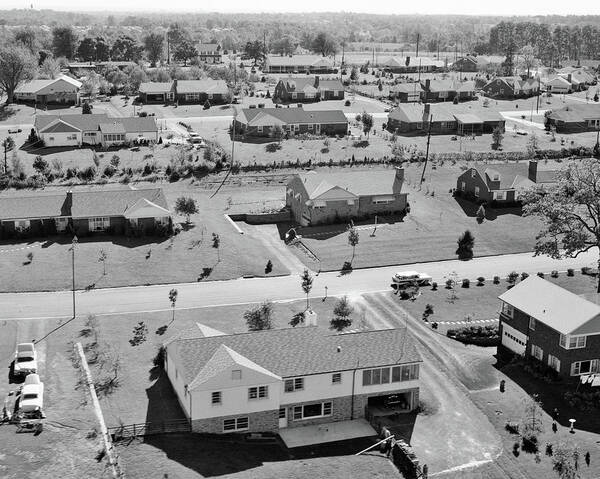This black-and-white aerial photograph captures a typical suburban neighborhood, likely from the 1960s or 70s, featuring a mix of two-story and ranch-style homes. Each house is spaced out, contributing to the overall sense of openness in the area. The streets appear quiet and lined with a few older model cars, including two white vehicles parked in the bottom left corner of the image. The neighborhood layout includes L-shaped clusters of homes and a backdrop of wooded areas beyond the residential lots. There are bushes in most of the yards and only one house with a white fence, while the majority of the properties have unfenced, open yards. The absence of modern amenities and text in the photo emphasizes its period style and serene atmosphere.